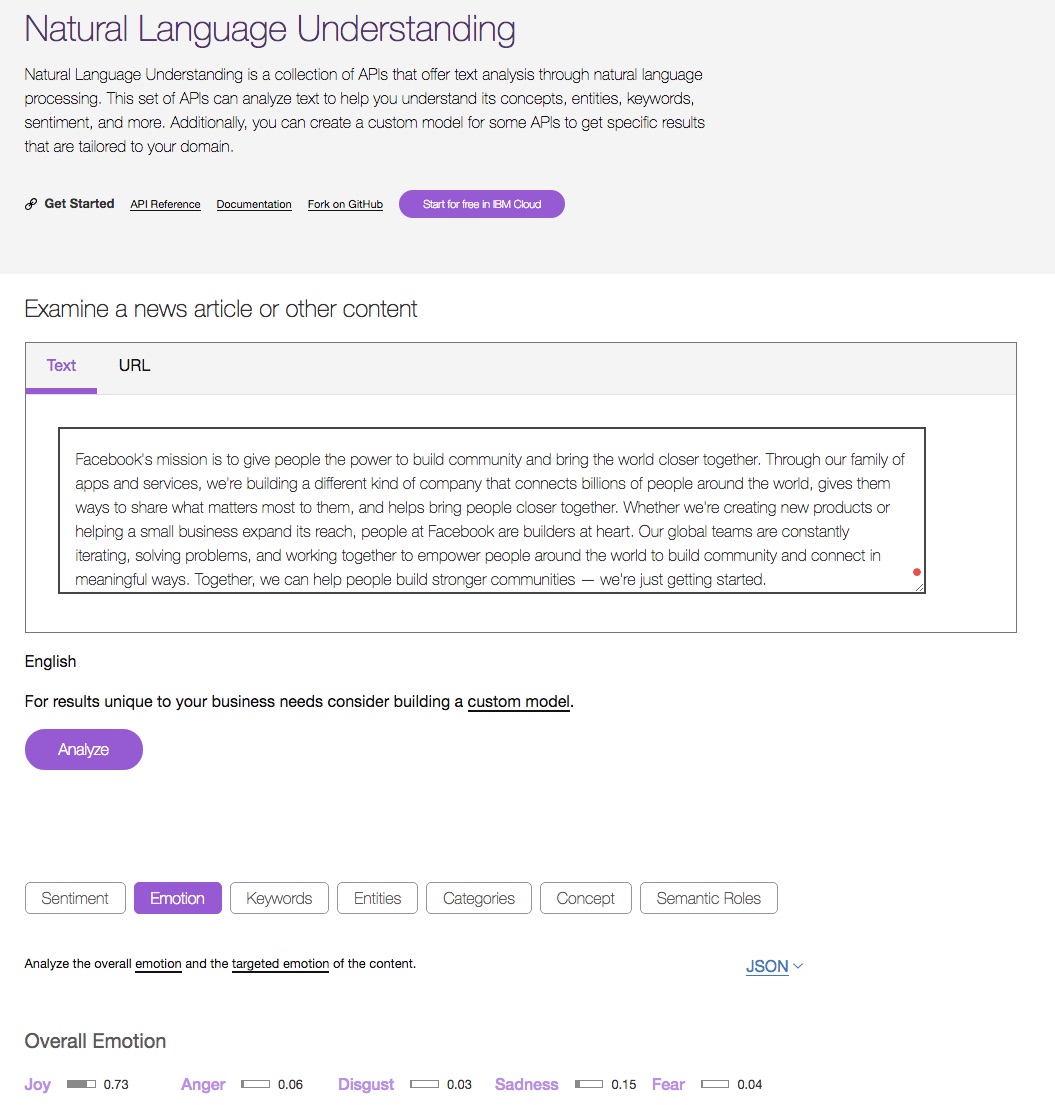The image features a screenshot set against a gray and white background. The top section of the image has a pale gray banner with dark lavender or dark purple text that reads "Natural Language Understanding." Below this, in smaller black text, is a description: "Natural Language Understanding is a collection of APIs that offer text analysis through natural language processing."

Underneath this description is a horizontal menu that includes several links. The first link is "Get Started," followed by "API Reference," which is underlined, indicating it is the currently selected option. The subsequent links are "Documentation" and "Fork on GitHub," with the latter also underlined. To the far right of the menu is a prominent purple action button that reads "Start for Free in IBM Cloud."

Below this banner, set against a white background, is a line of black text that instructs users to "Examine a News Article or Other Content." Beneath this directive, there is a gray box outlined in dark gray that contains the text: "Facebook's mission is to give people the power to build community and bring the world closer together."

At the bottom of the gray box is another purple action button labeled "Analyze," inviting users to proceed with text analysis.